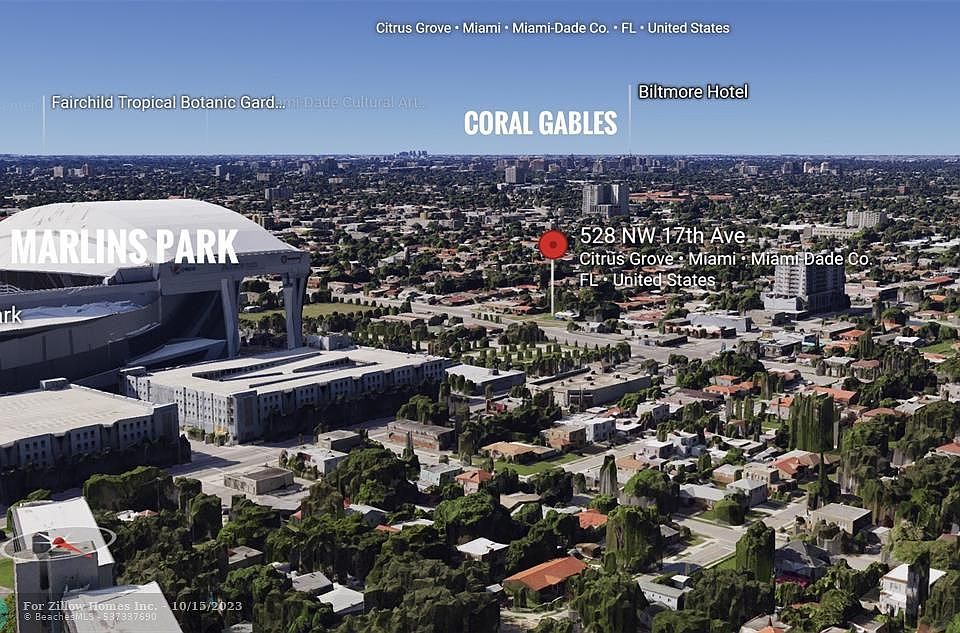The image is an aerial view, resembling a Google Earth snapshot, depicting a portion of Miami-Dade County, Florida, prominently focusing on Coral Gables. Multiple landmarks are clearly annotated with white lettering and directional lines, creating a detailed map-like representation. 

In the upper left-hand corner, the large dome of Marlins Park is labeled prominently. Slightly above that, "Fairchild Tropical Botanical Garden" is designated, with a guiding line indicating its location. Centrally placed at the top is the label "Citrus Grove, Miami, Miami-Dade County, Florida, United States," beneath which the "Biltmore Hotel" is marked with another directional line. 

The address "528 Northwest 17th Ave" is highlighted with a red pin icon, situated within the labeled area of "Citrus Grove, Miami, Miami-Dade County, Florida, United States." 

The landscape is a mix of gray tones from the streets, main avenues, and tall buildings, interspersed with patches of greenery from trees and bushes. The buildings predominantly feature red roofs amidst the graystone structures, extending out to meet the blue sky forming a strip across the top of the image.